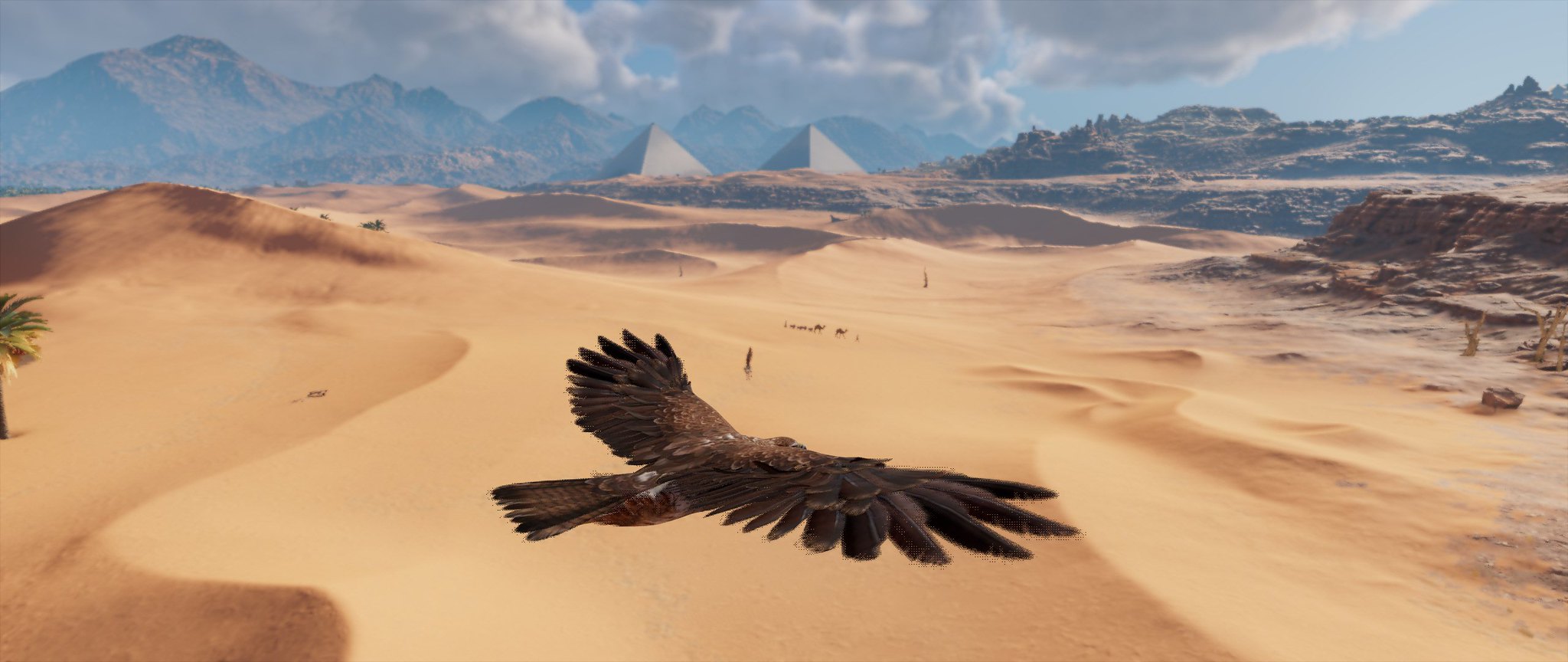The image is a highly detailed desert scene, potentially a computer-generated screenshot from a video game, showcasing a wide expanse of light beige and tan desert sands, subtly undulating with hills and valleys. Dominating the sky is a large brown bird, resembling a hawk or an eagle, with its wings majestically outstretched as it soars high above the terrain. In the middle distance, two pyramids crafted from sandstone rise prominently from the desert, with their shaded right sides contrasting against their sunlit left sides. To the far right, a half-visible palm tree adds a touch of greenery to the arid landscape. The background features a dramatic mountain range that ascends progressively higher towards the right, crowned by huge, white, and slightly stormy clouds. As you move towards the left, the sky transitions to a clearer, baby blue above smaller, browner hills. This atmospheric scene is illuminated by the ruminating sunlight, enhancing the overall shiny and pristine quality of the desert sands.